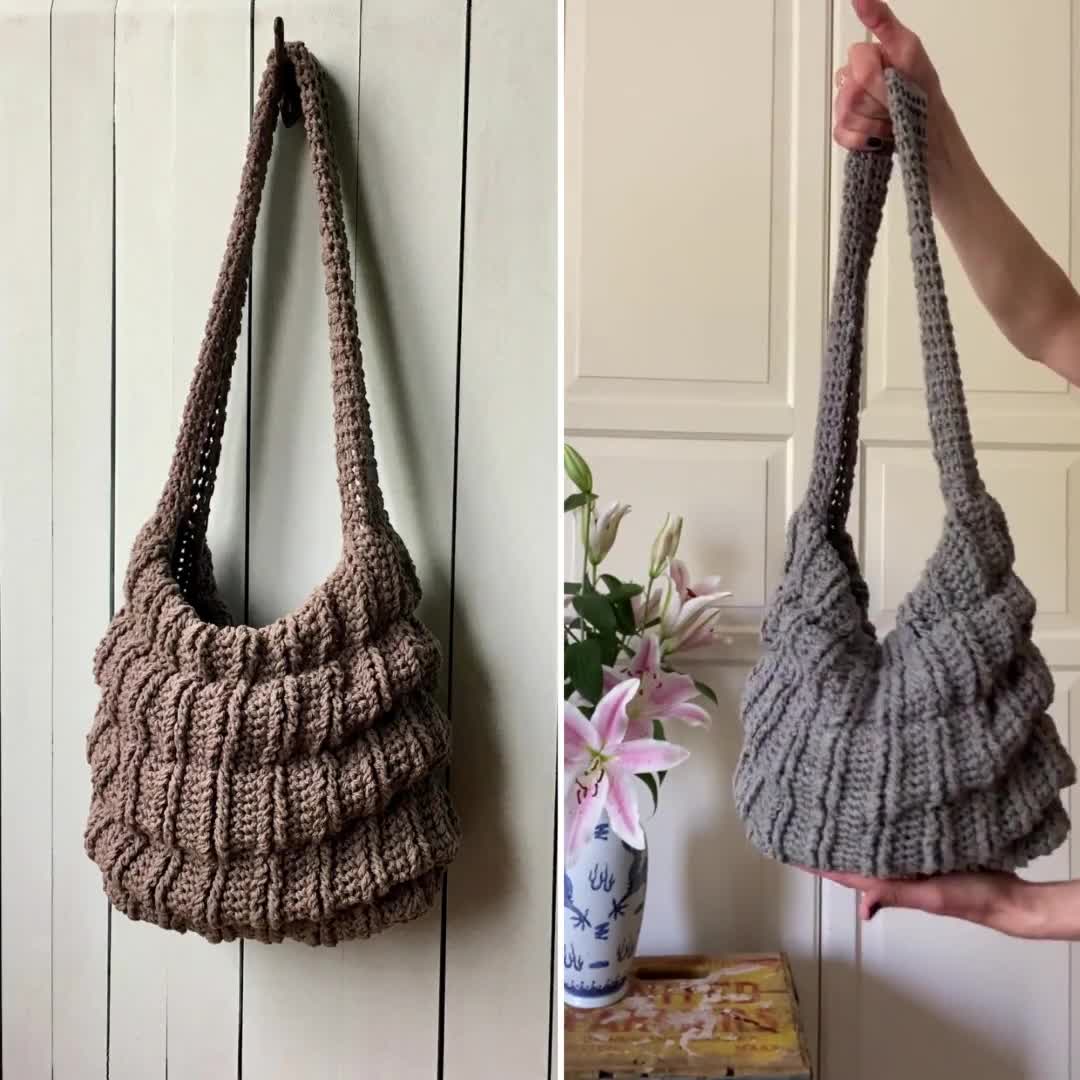In this side-by-side photo set, each oblong-shaped image showcases a beautifully crafted crochet or knitted purse. In the left image, the tan-colored purse hangs elegantly from a black hook mounted on a wall of white wooden slats. The purse itself is intricately designed with four distinct curved tiers, each interconnected, and embellished with vertical sets of double lines that run down its height, enhancing its textured appearance.

The right image contrasts by featuring a gray version of the same purse, now held by a person. One of their hands clutches the strap while the other is placed underneath, stabilizing the bag and better displaying its shape. The background reveals a serene setting with white-paneled cabinets, accompanied by a small table adorned with a blue vase filled with vibrant pink flowers, adding a touch of natural beauty to the composition.